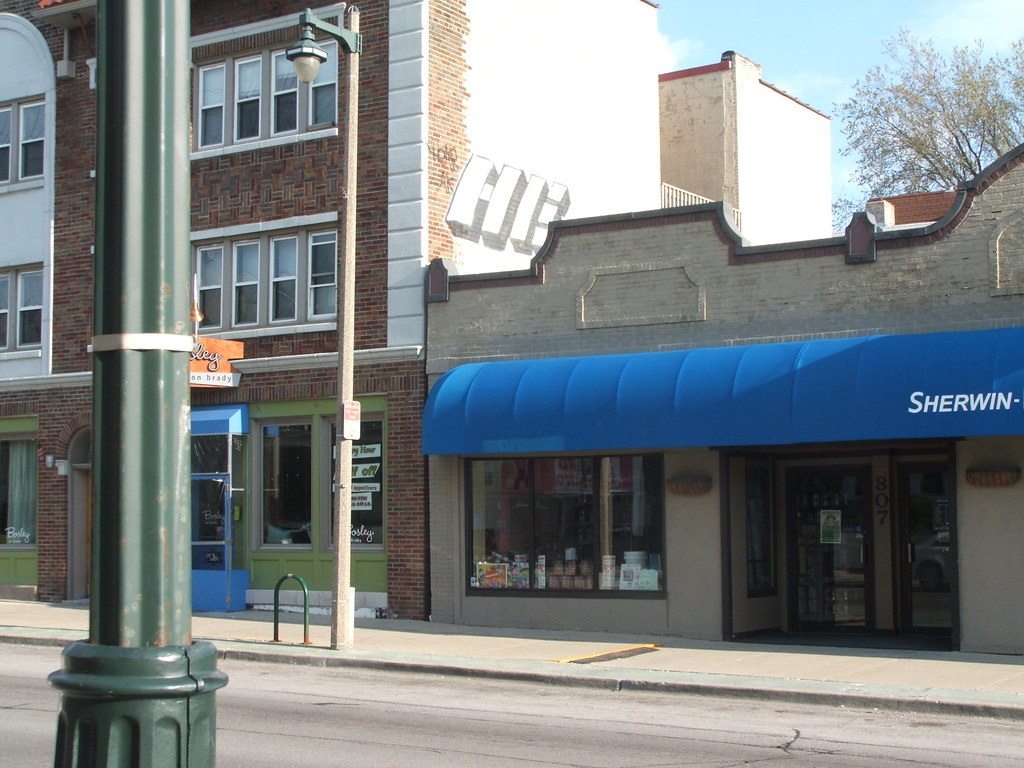This photograph captures a quaint small-town street scene featuring a mix of architectural details and storefronts. The central focus is on a Sherwin-Williams paint store, housed in a gray, one-story brick building with a prominent blue awning displaying the name "Sherwin" in white text. Below the awning, a door with a black frame and adjacent windows showcase paint products. To the left of the Sherwin-Williams store stands a three-story brick building with red bricks and green-painted architectural elements around the windows and doorways. The ground floor hosts additional, yet unidentified, storefronts with tall, thin rectangular windows on the upper floors. In the left foreground, a dark green metal telephone pole stands out against the street. Off to the right, the background reveals a sparse tree and a clear blue sky, adding a touch of nature to this charming street scene.